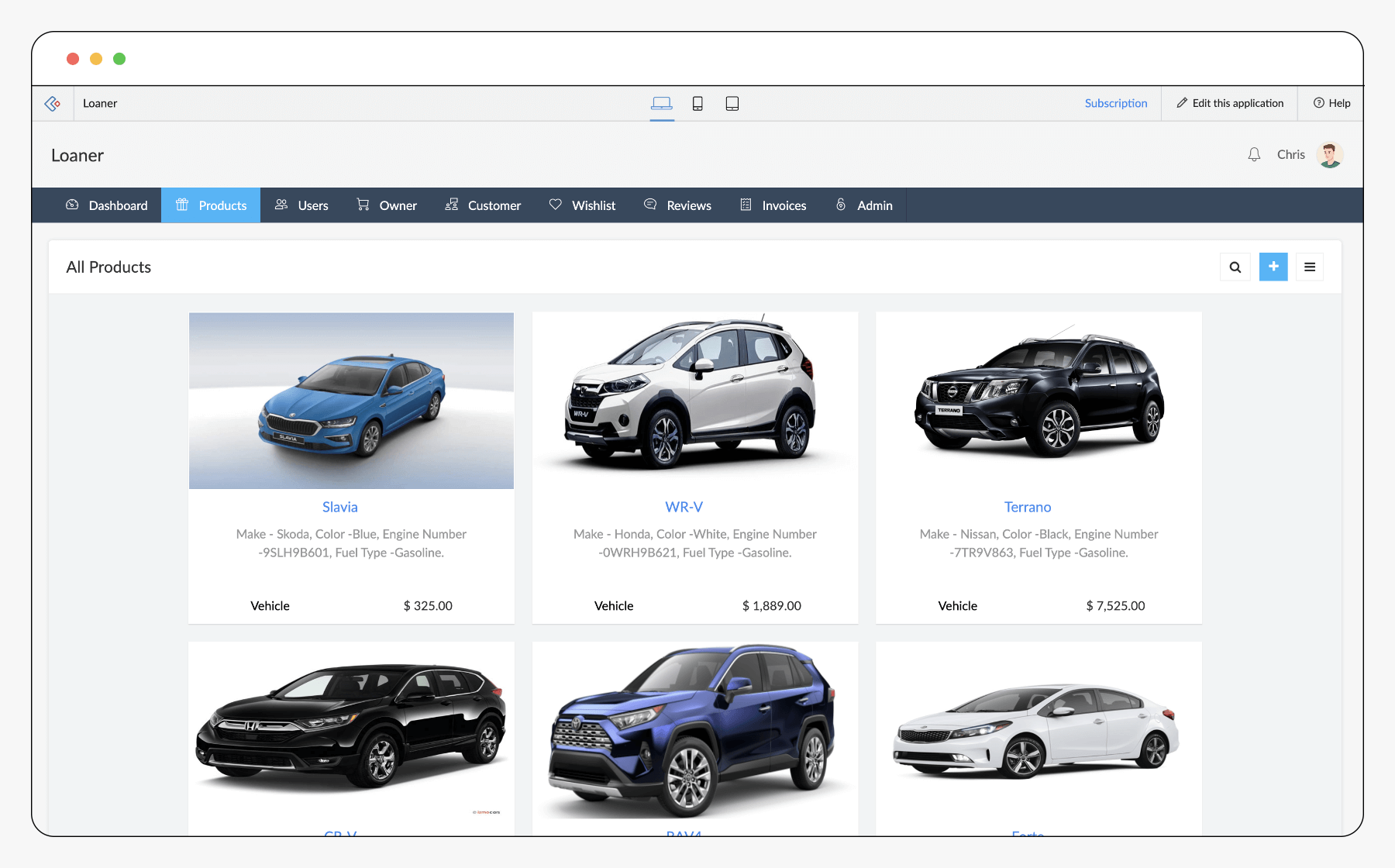In this image, you see a webpage from the Luna website, which features a detailed dashboard interface displaying vehicles and their prices. At the top of the page, various sections are linked, including Dashboard, Products, Users, Owner, Customer, Wishlist, Reviews, Invoices, Admin, and All Products.

The main content area showcases a range of vehicles with specific details for each. One featured vehicle is the Slavia, identifiable by its blue color and engine number, with a vehicle price listed at $325. Another vehicle displayed is the WRV, a white Honda, noted for its vehicle loan price of $1,889. Further down, the Terrano, a black Nissan, is presented with a vehicle loan price of $7,535.

Additionally, the image reveals there are three other cars listed below these main entries. Another noteworthy detail includes the roofing costs displayed prominently at $14,000. The overall interface appears user-friendly, providing comprehensive information about the vehicles available on the Luna platform.